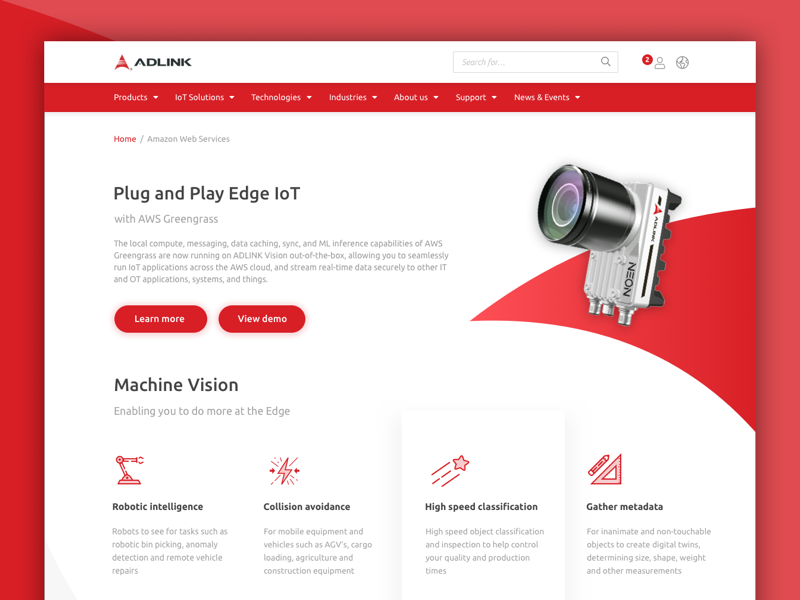**Screenshot of Adlink Web Page: A Detailed Overview**

The screenshot captures the web page of Adlink, a company with a distinctive red logo resembling an upward-pointing arrow curved at the bottom, positioned to the left of the word 'Adlink'. At the top of the page, a search bar is prominently displayed. To the right of the search bar are icons indicating user notifications (showing the number 2), a people icon, and a globe icon.

Below this section, a horizontal red banner stretches across the page, featuring pull-down menus labeled as follows: Products, IoT Solutions, Technologies, Industries, About Us, Support, News and Events.

Continuing down the page, you see breadcrumb navigation reading "Home / Amazon Web Services" on the left side. On the right side, there is an image of a camera, showcasing a sturdy silver casing with a sizable lens and several connection ports at the bottom.

Text accompanying the camera image reads, "Plug and Play Edge IoT with AWS Greengrass." It further explains, "The local compute, messaging, data caching, sync, and ML inference capabilities of AWS Greengrass are now running on Adlink Vision out-of-the-box, enabling seamless IoT application deployment across the AWS cloud and secure real-time data streaming to various IT and OT or DT applications, systems, and devices." Adjacent to this text are two red buttons labeled 'Learn More' and 'View Demo'.

Below this content, the heading "Machine Vision" is prominently displayed, followed by the subheading "Enabling you to do more at the edge." The section highlights four key topics: 

1. **Robotic Intelligence**: Described as "Robots that see for tasks such as robotic bin picking, anomaly detection, and remote vehicle repairs."
2. **Collision Avoidance**: Explained as "Solutions for mobile equipment and vehicles such as AOVs, cargo launching, agriculture, and construction equipment."
3. **High-Speed Classification**: Detailed as "High-speed object classification and inspection to improve control over production times and quality."
4. **Gather Metadata**: Outlined as "For inanimate and non-touchable objects, enabling the creation of digital twins and the determination of shape, weight, and other measurements."

This comprehensive screenshot provides a clear and detailed view of Adlink's web page content, prominently showcasing its IoT and machine vision solutions integrated with AWS Greengrass.